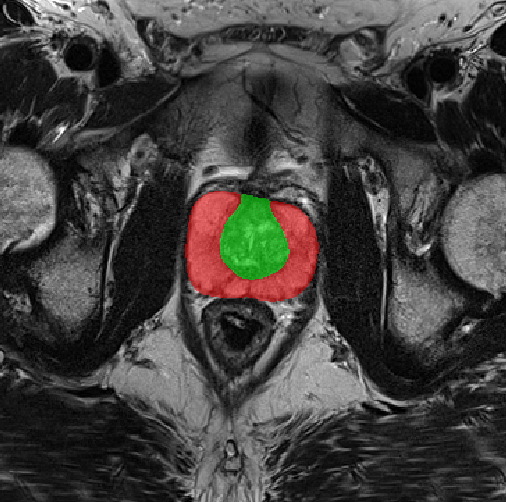The image appears to be a zoomed-in MRI or x-ray of the internal organs of an unidentified creature. The primarily black and white image showcases various tube-like and muscular structures dispersed throughout, with a particular focus on the bottom left and right areas where muscle tissues are discernible. Encircling a highlighted area are fatty tissues. This highlighted section stands out due to specific coloring: a central white area, overlaid with green, and surrounded by a red horseshoe-shaped band. The image's abstract quality gives it an almost art-like appearance, with a notably dark, nearly black background interspersed with white dashes, creating an impressionistic feel. Overall, the colored central region contrasted against the monochrome background emphasizes the peculiar focal point of the image.